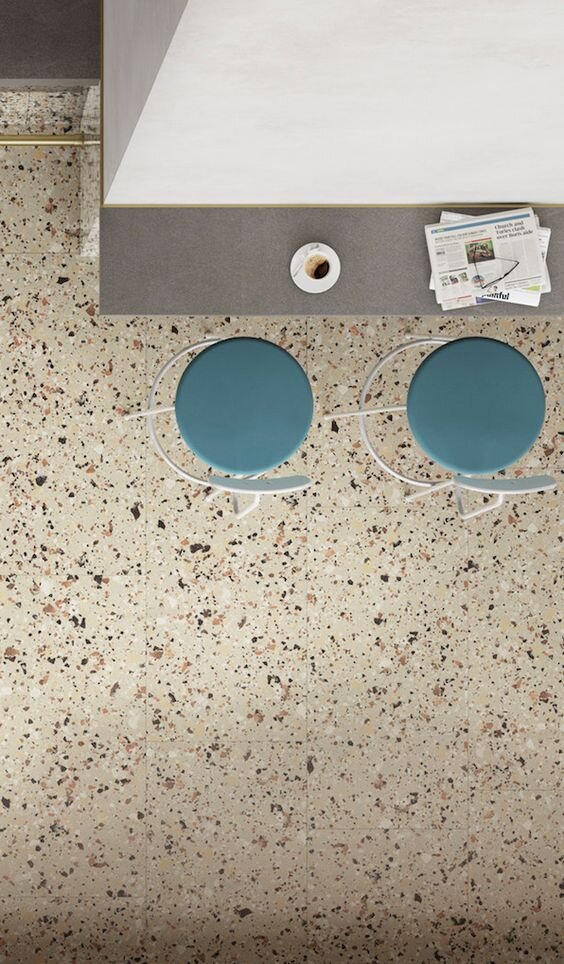This image is an aerial view of a quaint cafe setting. At a bar-height ledge, two teal bar stools with white backrests are positioned closely together, inviting company. The ledge, possibly made of gray material, extends from a wall, serving as a makeshift bar. Resting on this ledge are a steaming cup of coffee and a neatly folded newspaper, with a pair of reading glasses placed on top, suggesting someone’s momentary departure from their morning reading ritual. The floor, depicted with a marbled brown stone design, adds a touch of rustic charm to the scene. A subtle shadow casts over the left side of the table, adding depth and a hint of mystery to the cozy environment.